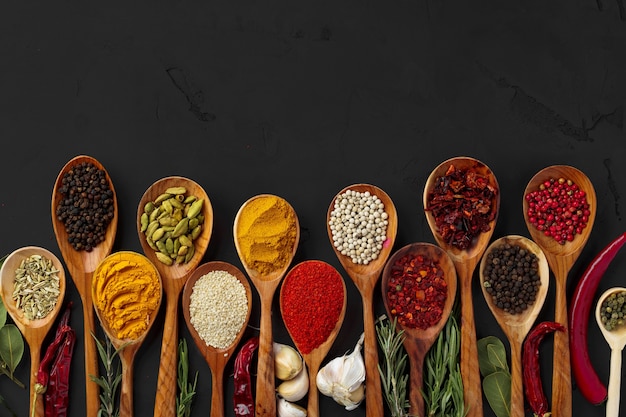The image features a striking dark gray, matte background with two rows of wooden spoons prominently arranged. Each spoon, extending from the bottom of the frame, is filled with a different vibrant spice. In the bottom row, there are six main wooden spoons and a smaller white one, all containing varied spices such as turmeric, peppercorns, green pumpkin seeds, and chili flakes. The top row also features six wooden spoons, similarly filled with a diverse array of spices and seasonings. Scattered among the spoons are additional aromatic elements, including garlic cloves, rosemary sprigs, and what appear to be sun-dried tomatoes, creating a rich and evocative display of culinary ingredients.